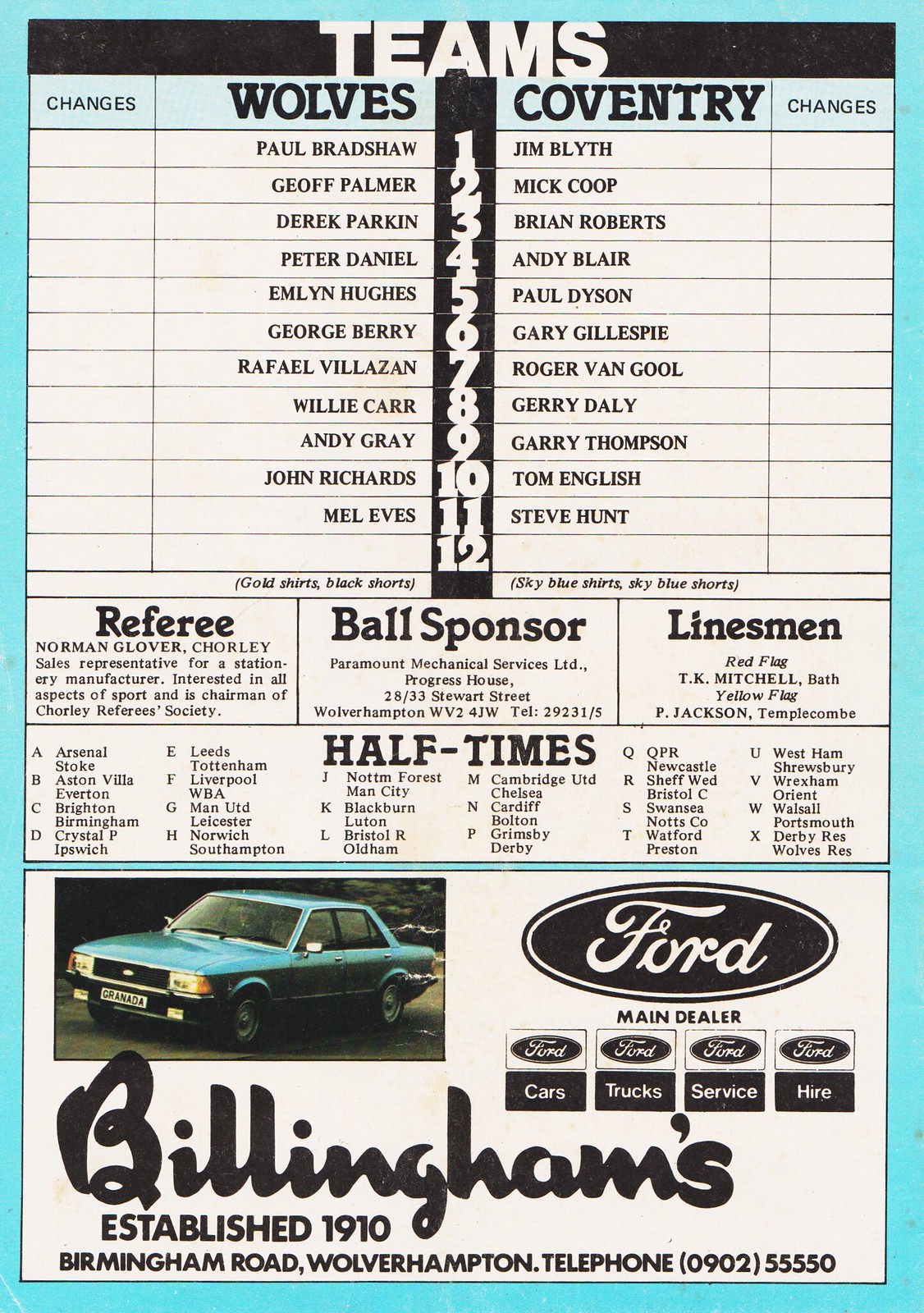This image displays a page from a soccer publication that appears to be a soccer pamphlet or program. The page is bordered by a blue and teal outline, framing its off-white background. At the top, there's a section titled "Teams" listing the squads for two teams: Wolves and Coventry. Each team roster includes 11 names arranged side by side, with the numbers 1 through 12 running down the center between them. Below the team rosters are three rectangular boxes labeled "Referee," "Ball Sponsor," and "Linesman," each box providing pertinent information.

Further down is a long rectangular box titled "Half Times," which presumably lists different teams. At the very bottom of the page is an advertisement featuring a vintage turquoise car, likely from the 1980s or earlier. This car is part of an ad for Billingham's Ford dealership, which includes the Ford logo and phrases like "Ford Cars, Trucks, Service, Hire." Additionally, there is a cursive logoed signature that reads "Billingham's, Established 1910, Birmingham Road, Wolverhampton, Telephone Number."